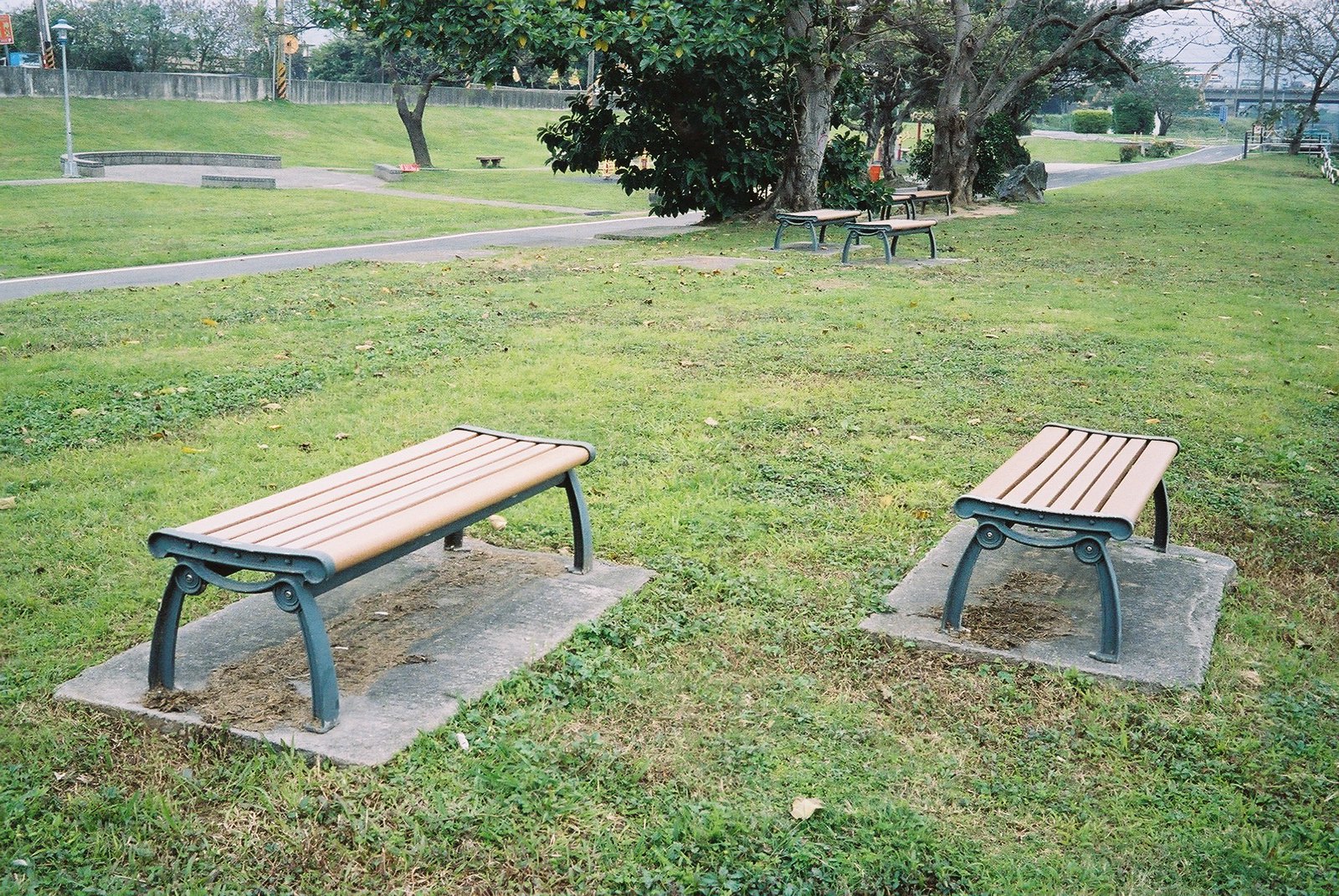The image depicts an outdoor park scene with two prominent backless benches in the foreground, one a single-seater and the other a double-seater. Both benches are placed on light gray concrete pads, surrounded by patches of dry leaves. The benches have dark green legs and corners with light brown plastic seating. Further into the background, similar benches can be seen, also situated on concrete pads between two large trees. A concrete walking path runs across the scene, and in the background, a partially visible overpass is bordered by trees and bushes. To the left, there is a stone wall with additional trees. On the right side, a circular concrete pad with a low wall that appears to be seating, and a light pole mark the area, near which a chain link fence and a bridge are faintly visible. The entire area is grassy with interspersed leaves, adding to the serene park atmosphere.